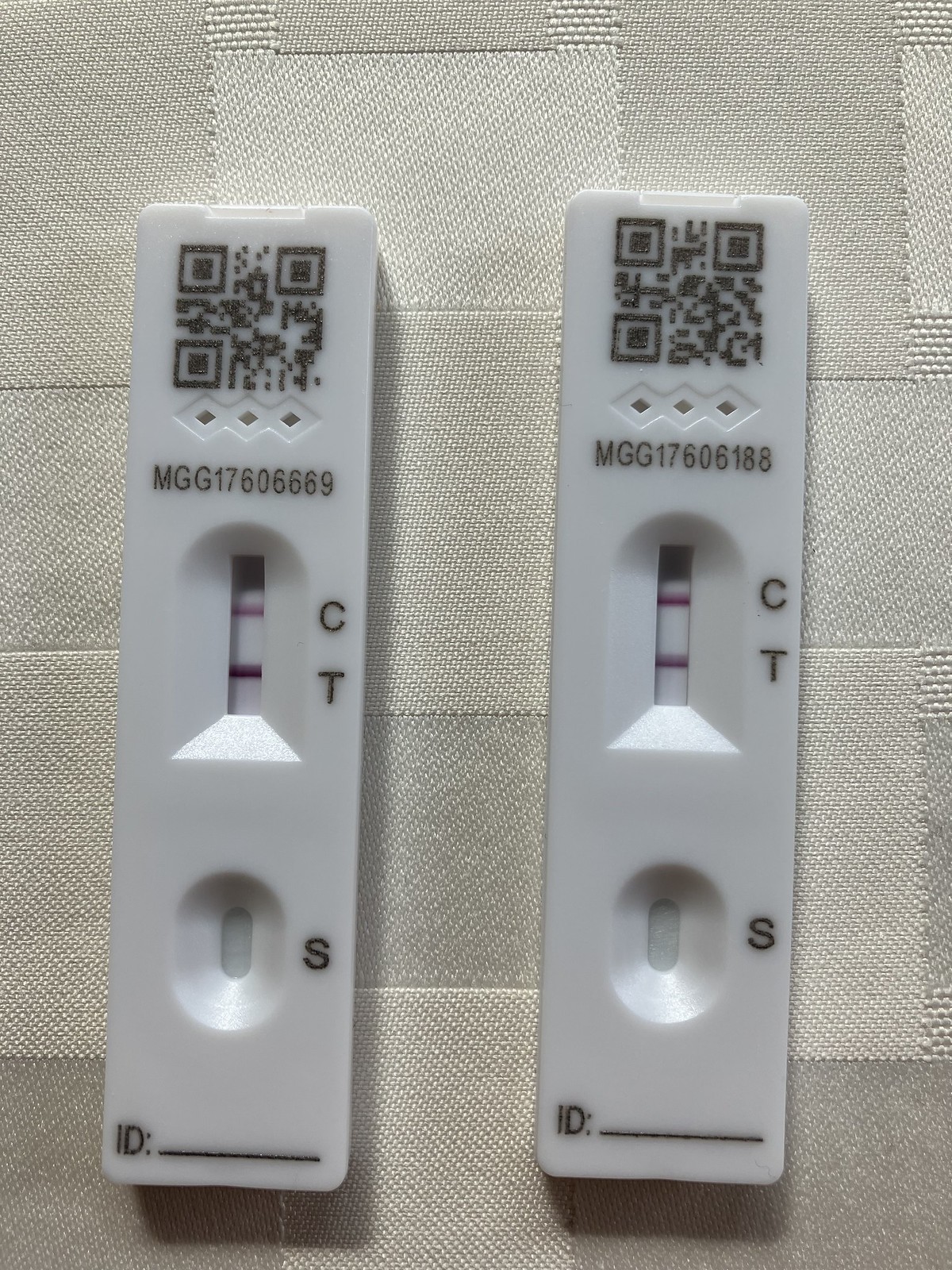This photograph shows two COVID-19 rapid tests placed vertically on a white cloth with a quilted pattern featuring white and gray squares. Each test has a small, square QR code at the top, followed by three triangular icons and a unique identifier number—for example, "MGG 176." The tests are clearly labeled with "C" for the control line and "T" for the test line. 

The test on the left displays a light purple control line and a dark purple test line. Towards the bottom, an area marked "S" is visible where the sample drops are placed through a small hole. An "ID" line at the very bottom is available for labeling the test with a name or identifier. 

Similarly, the test on the right is nearly identical in layout. It features a different unique identifier number and shows a darker purple control line and a lighter purple test line. Each component, from the QR code to the "ID" field, mirrors the design of the test on the left.